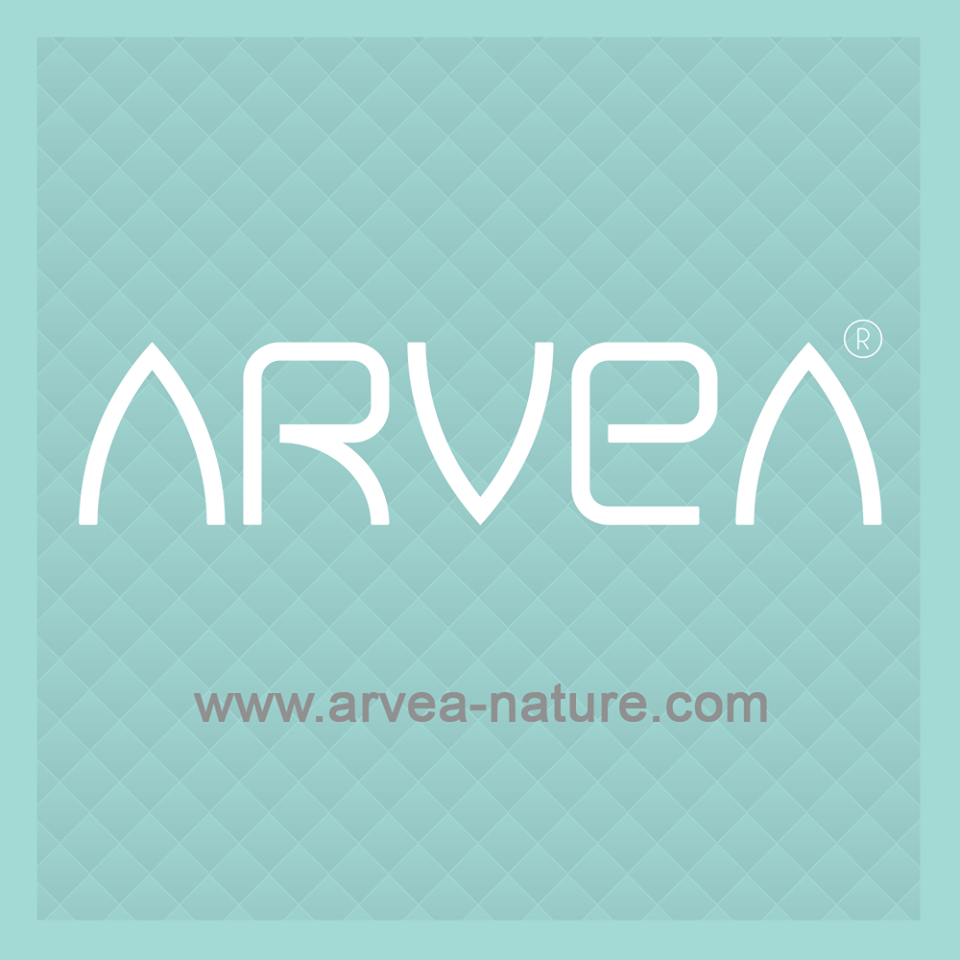The image is a vertical, moderately wide rectangle featuring a pale teal blue background with a pattern of small triangles or diamonds. The border trim around the edges is a solid light teal blue. Across the center, in large white capital letters, the text "ARVEA" is prominently displayed, accompanied by a trademark symbol (a capital R in a circle) slightly to the upper right. Below this, in a dull black or dark gray color, the website "www.arvea-nature.com" is written, positioned just above the bottom part of the image. The overall design seems like a promotional sign for Arvea, possibly a screenshot of a website or digital advertisement.